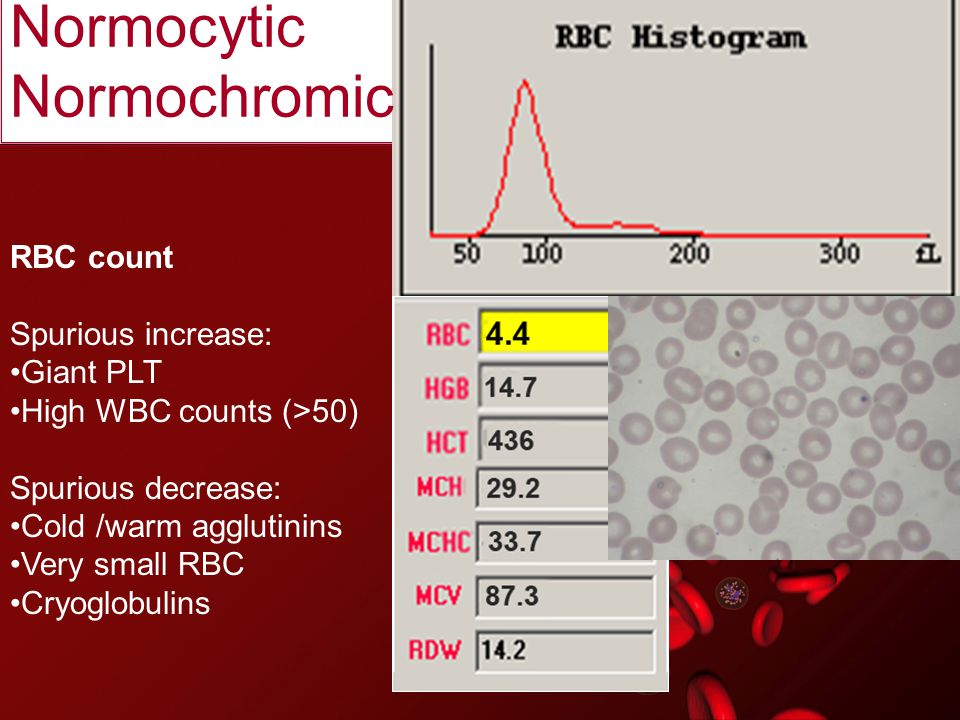This is a computerized graphic with an educational focus, likely from a PowerPoint presentation on hematology. The slide features a predominantly red background with white text, emphasizing information about Red Blood Cells (RBC). In the upper left corner, the title "Normocytic, Normochromic" is displayed. Below, in white text on a deep red background, the section "RBC count" is divided into subsections. "Spurious Increase" includes bullet points for "giant PLT" and "high WBC counts > 50." "Spurious Decrease" lists three bullet points: "cold/warm agglutinins," "very small RBC," and "cryoglobulins."

On the right side, a chart titled "RBC histogram" shows a red line graph with an x-axis labeled possibly in fluid liters and marked at 50, 100, 200, and 300. Below this, another chart itemizes values for RBC, HTB, HTC, among others, with figures like 4.4, 14.7, 4.3, and 6, highlighted in gray and one in yellow. In the lower right corner, there is an image of various blood cells. Altogether, this slide integrates text, charts, and graphs pertinent to medical professionals analyzing red blood cell counts and related data.